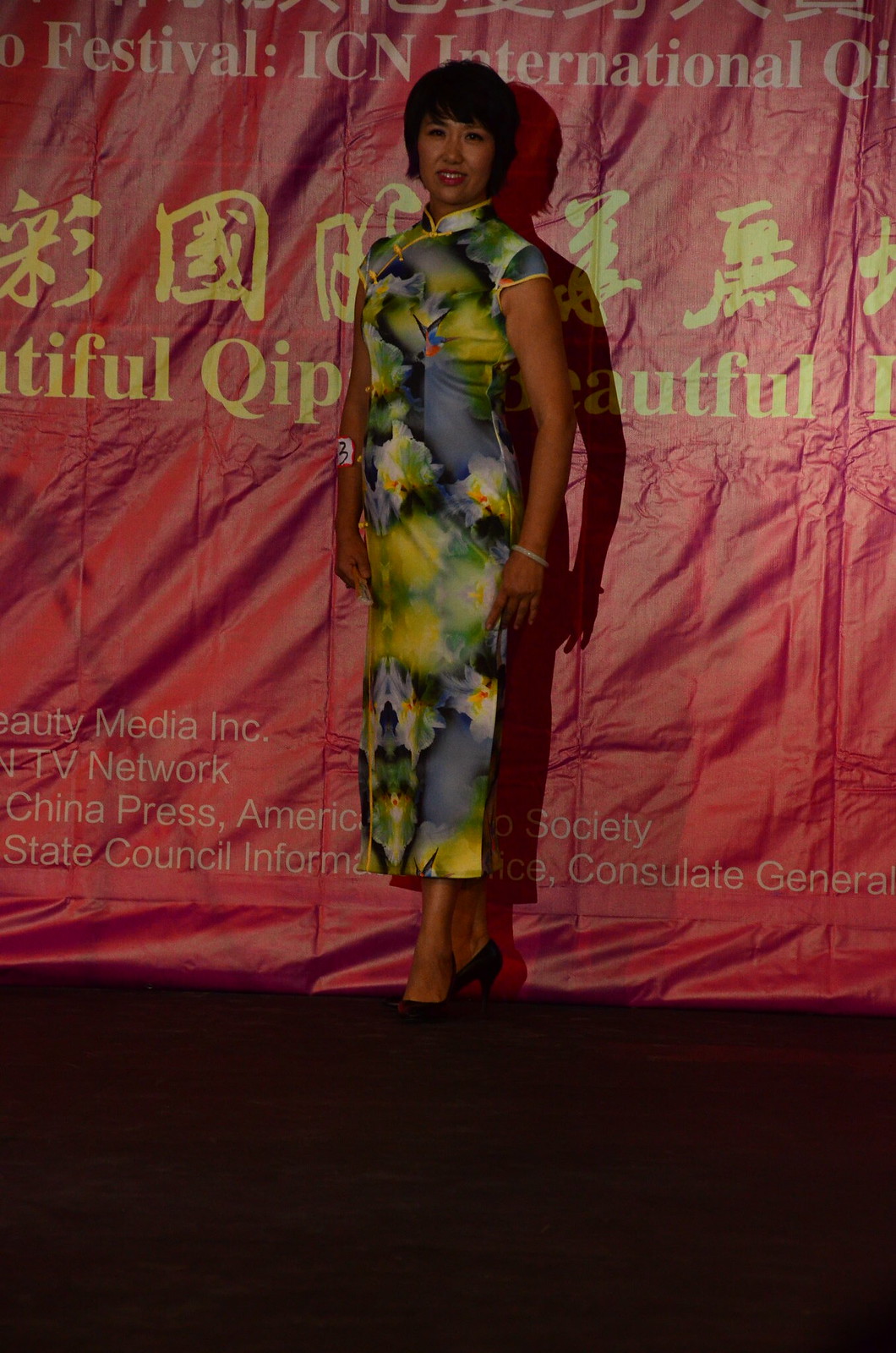A woman, who appears to be Asian, is posing in front of a large red banner that partially obscures the text, though "Festival ICN International" and some Chinese characters can be discerned. The banner also features text referencing "TV network, China Press, America." The woman is dressed in a form-fitting, traditional Chinese dress which is adorned with a vibrant fusion of yellow, green, gray, and black colors. The dress features a distinctive floral design interspersed with red, blue, and black birds that resemble swallows. She has short, above-the-shoulder black hair with bangs swooshing to the right. The high collar of her dress is accentuated by a yellow hem and three buttons extending from the leg area down to the right side of her chest. She is smiling and also wearing a jade bracelet on her left wrist, which adds a touch of elegance to her ensemble. The backdrop and her poised demeanor suggest that the photograph might have been taken at a formal event, possibly a press photo area.